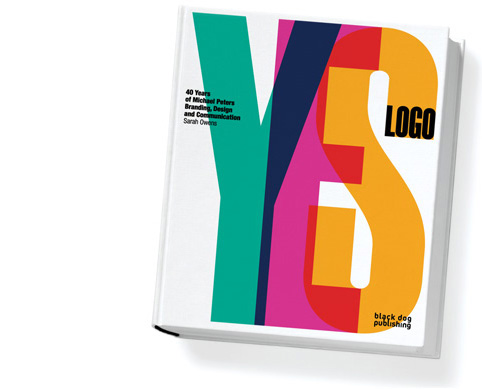This photograph showcases a book isolated against a white background, featuring a minimalistic yet colorful cover design. The cover prominently displays the word "YES" in an overlapping typography that beautifully merges colors where letters intersect. The letter 'Y' is a vibrant teal green, overlapping with a pink 'E,' transitioning into orange where they intersect. The 'Y' also appears with a navy blue left upward arm where it overlaps the 'E'. The 'E' further overlaps with a yellow 'S', turning pink into orange at their intersection. The letter 'S' is yellow and has "LOGO" written in bold black capital letters at the top part of its curve. In the upper left corner, there is a block of black text in bold, detailing "40 years of Michael Peters branding, design, and communication," followed by the name "Sarah Owens," though this text is too small to discern specifics. The lower right corner features black lowercase text that reads, "Black Dog Publishing," just overlapping the bottom of the 'S'. The book casts a slight shadow at the right side and lower edge, indicating the light source is from the upper left. The overall composition adheres to a photographic realism style, emphasizing the clean, graphic design of this square-format book cover.